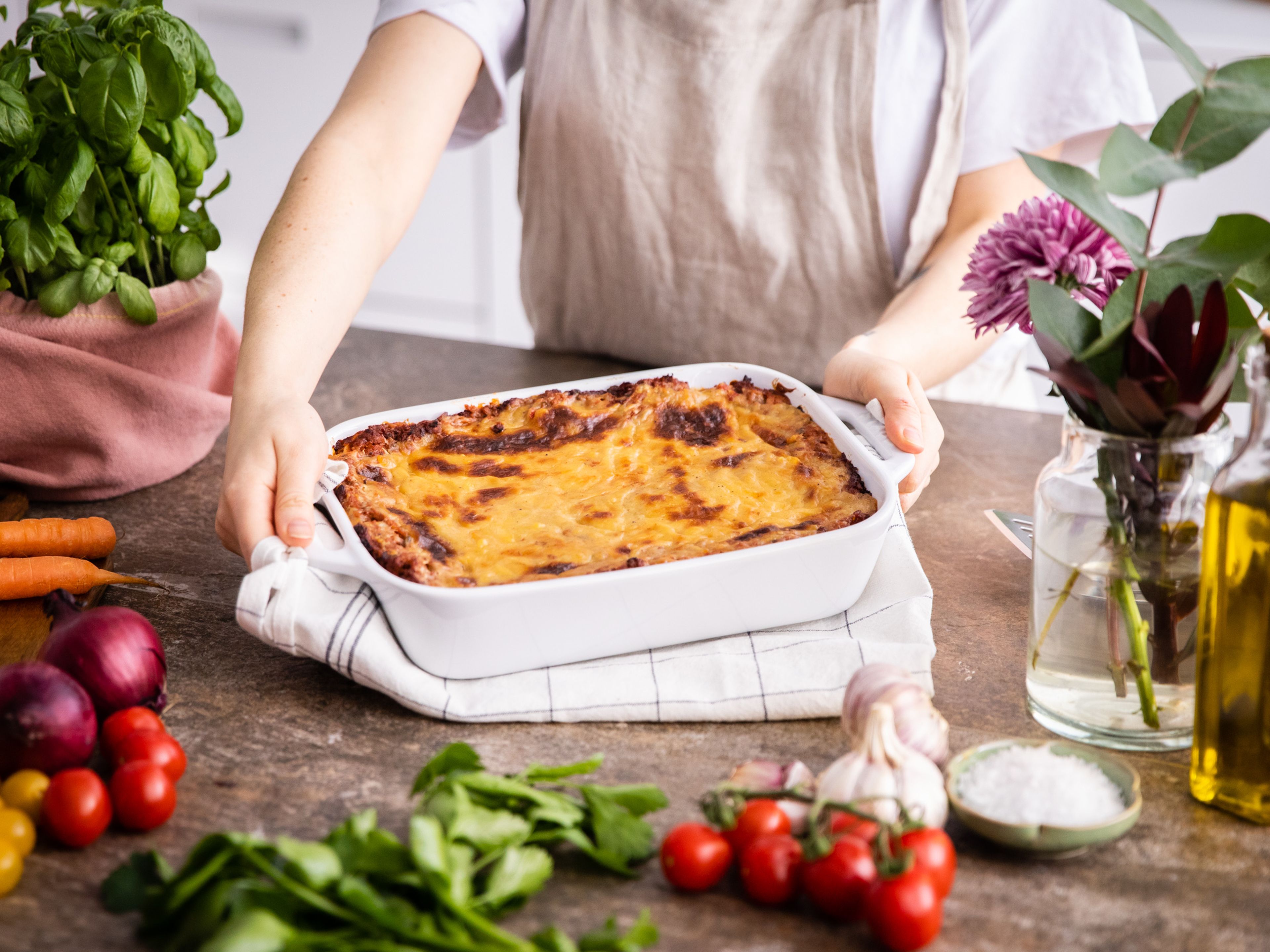In this detailed image, a person, visible only from their shoulders down, is standing over a rustic marbled brown countertop. They are dressed in a white t-shirt under a beige apron and are holding out a white ceramic baking dish, which sits on a folded white dishtowel. The dish appears to contain a golden-brown casserole, with some browned spots on the top, suggesting it might be lasagna or a similar baked dish. Surrounding the dish on the countertop are various fresh vegetables, including tomatoes, garlic, red onions, and carrots, as well as a small basil plant on the left. On the right side, there's a vase filled with flowers and a bottle of olive oil, contributing to the overall rustic and inviting cooking scene.